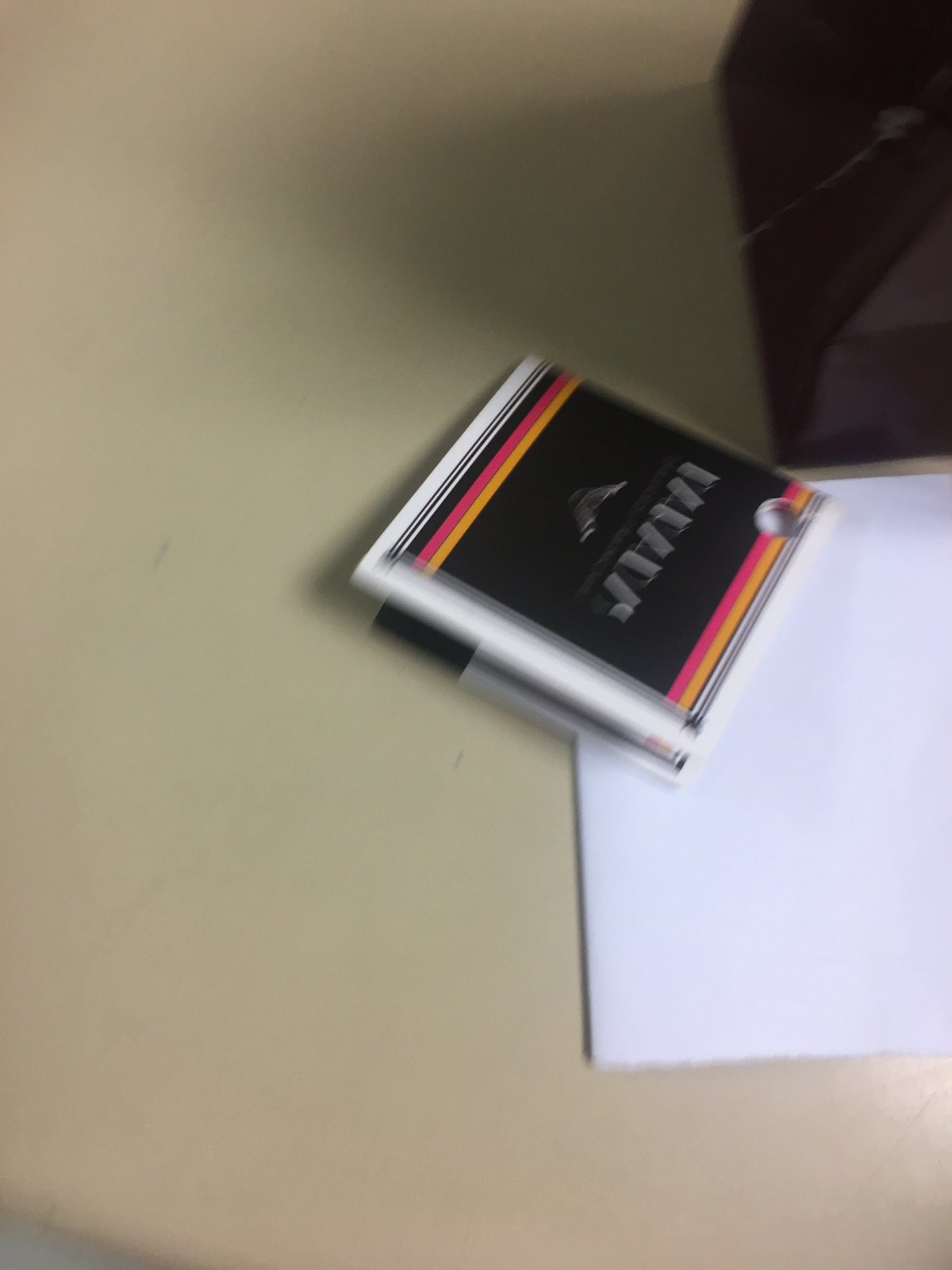A blurred, vertically oriented photograph showcasing a beige countertop or tabletop. In the upper right corner, there is a partially visible black object. Along the right edge, a white folded piece of paper extends towards the center of the frame. Near the center of the image lies a detached clothing tag, predominantly black with a white border and featuring horizontal bars in black, red, and orange at the top and bottom. The tag is rotated such that its bottom edge points towards the upper left corner, while the top edge angles towards the right center of the image. A hole is punched in the tag's upper left corner (appearing as the upper right in the image), indicating its previous attachment to a purchased item.